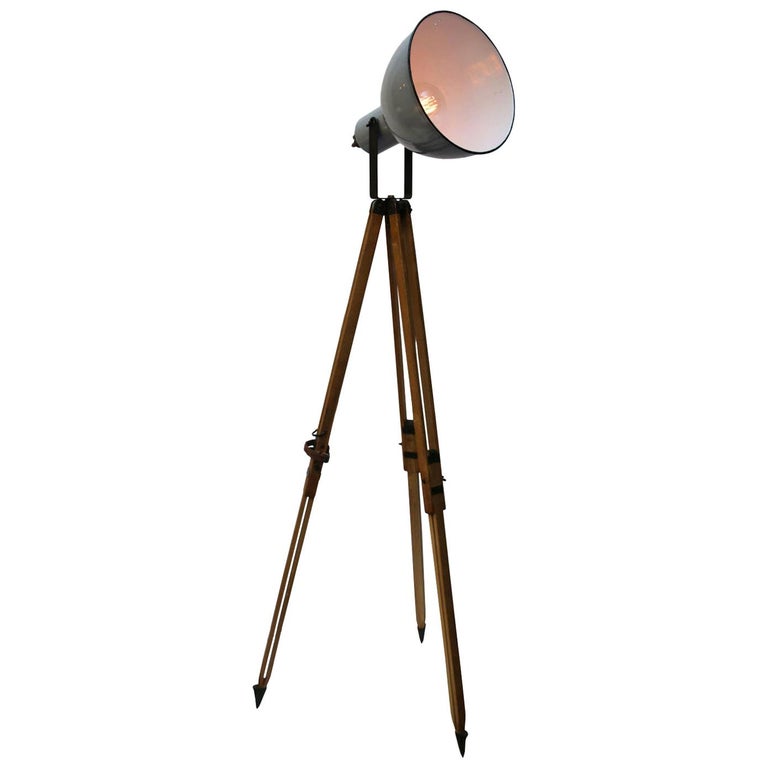This image features a detailed studio light mounted on a wooden tripod with a clean, white background. The studio light is encased in a sleek, black metal housing with a contrasting white interior that enhances the glow of the visible yellow light bulb inside. The black exterior contrasts sharply with the brown wooden tripod, whose extendable and collapsible legs are pointed at the ends with black tips. Positioned upright and aimed slightly upward, the studio light is configured as if to illuminate a scene for filming or photography, devoid of any additional context or surroundings, making it a striking and professional-looking piece of equipment.